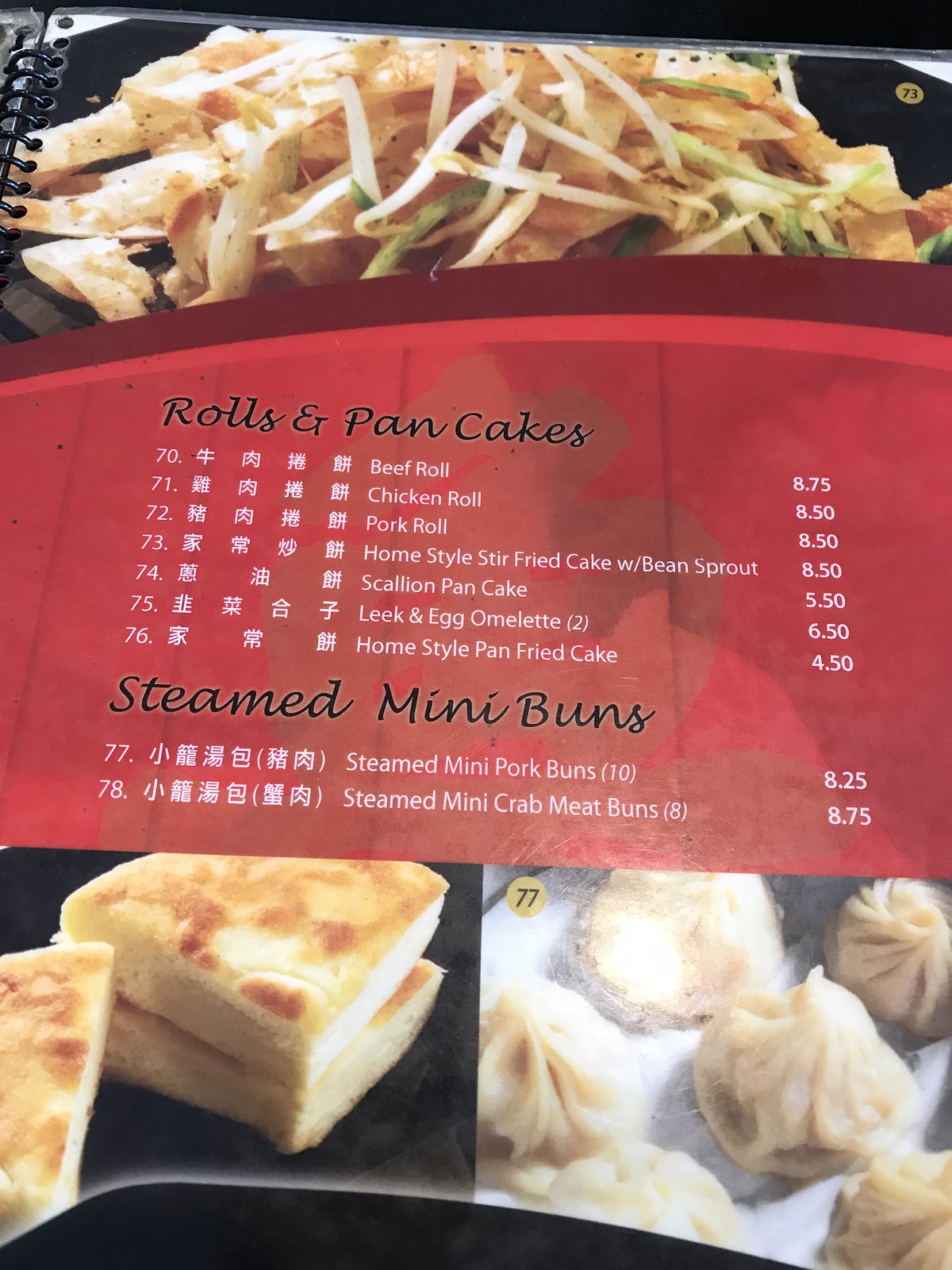The image features a multi-page menu, as indicated by the black ring spiral binding visible on the left side of the frame. The specific page in view highlights various food items, with a distinct yellow circle marked with the number "73" in the top right corner. Adjacent to the circle is an image of a dish that appears to be light brown noodles garnished with green sprouts.

The menu itself is presented against a red background, with the dish names listed in a cursive font. The section titled "Rolls and Pancakes" is numbered from 70 to 76 and includes both Chinese characters and English translations:

- Beef Roll: $8.75
- Chicken Roll: $8.50
- Pork Roll: $8.50
- Homestyle Stir-Fried Cake with Bean Sprout: $8.50
- Scallion Pancake: $5.50
- Leek and Egg Omelette (2): $6.50
- Homestyle Pan-Fried Cake: $4.50

Beneath this section, in black cursive font, items 77 and 78 are listed under "Steamed Mini Buns" with corresponding Chinese and English text:

- Steamed Mini Pork Buns (10): $8.25
- Steamed Mini Crab Buns (8): $8.75

The lower part of the image features photographs of dumplings on the right and a type of bread item on the left, further illustrating the culinary offerings.